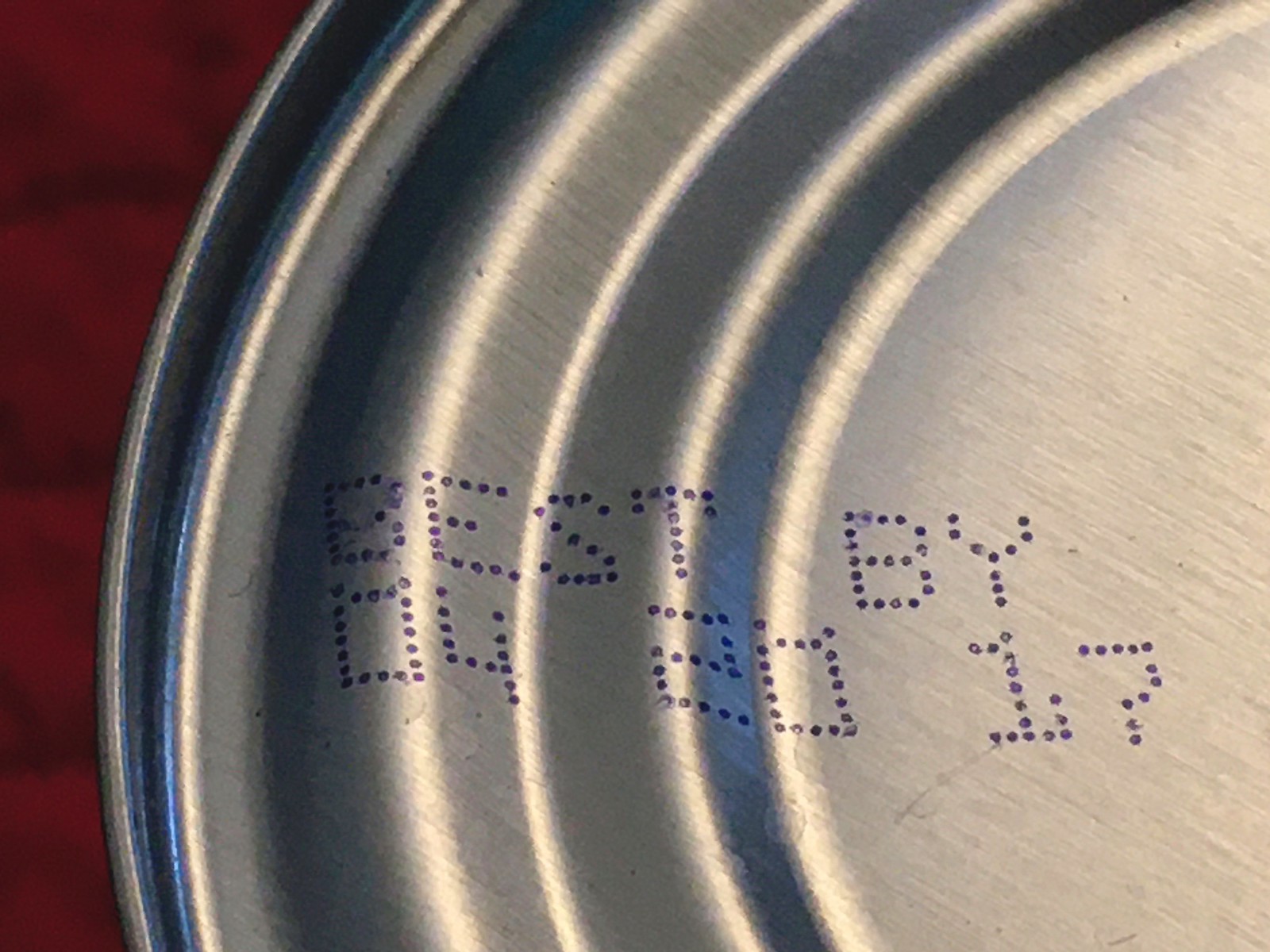This image is a horizontal macro photograph, capturing an extreme close-up of what appears to be the bottom of a silver, possibly aluminum, tin can of food. The can features multiple concentric rings or raised rims around its edge, creating a series of layered, circular patterns. Prominently stamped in the center of the can's bottom, formed by tiny purplish-blue dots, is a "Best Buy" date reading "04-2017," indicating the product's expiration date. The background on the left side of the image is blurry with a hint of red, providing contrast to the metallic surface of the can. The overall scene is somewhat dark, emphasizing the detailed texture and text of the can's bottom.